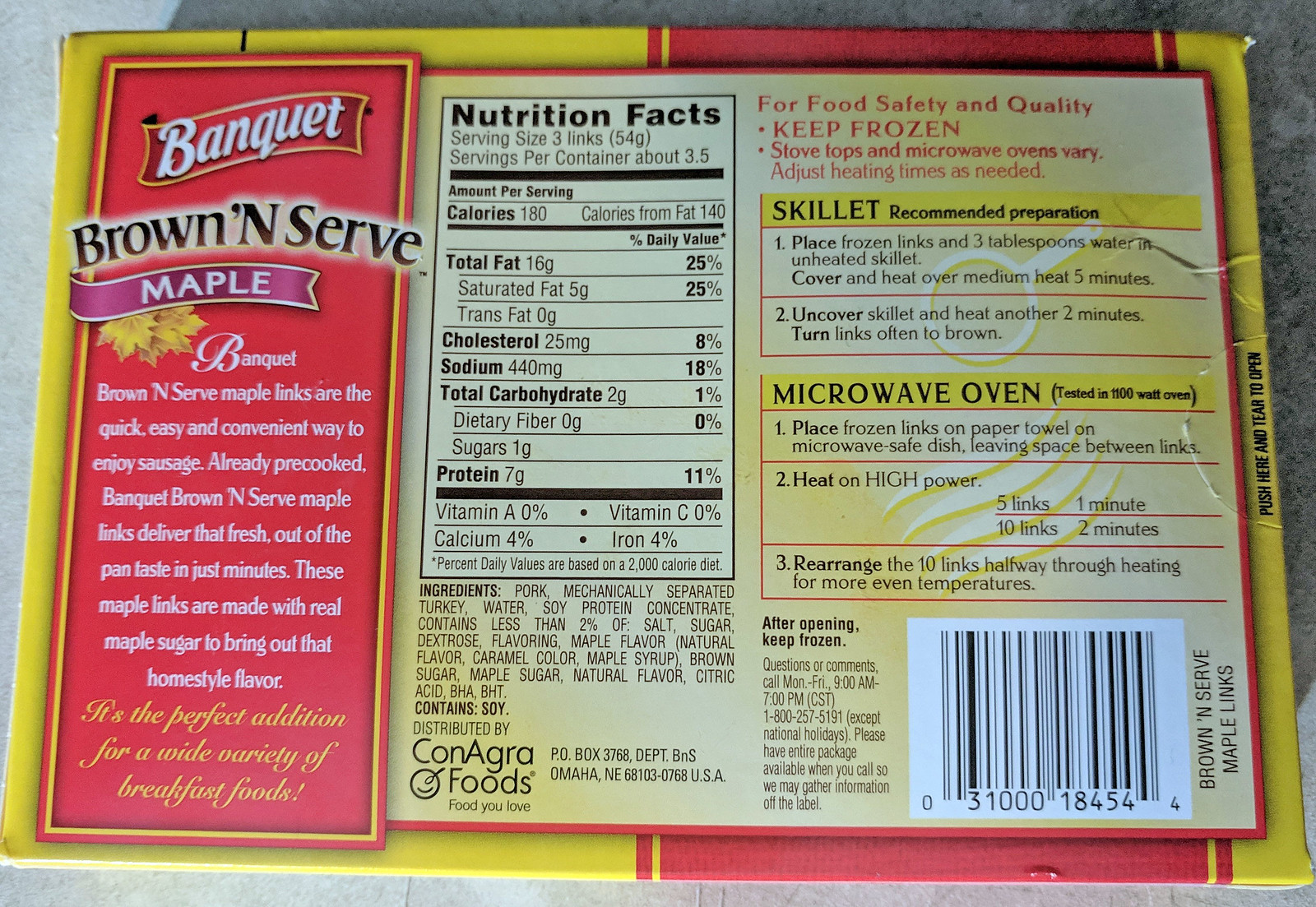The image depicts the back of a Banquet Brown and Serve Maple Sausage Links package. The package is square-shaped and primarily features a red and yellow color scheme. Dominating the left side is a red rectangle with a yellow outline that prominently states "Banquet Brown and Serve Maple Links." This rectangle includes text detailing that these pre-cooked sausage links are a quick, easy, and convenient way to enjoy sausage, delivering a fresh out-of-the-pan taste in just minutes. Made with real maple sugar, these links provide a homestyle flavor and are an ideal addition to a wide variety of breakfast foods.

The back of the box also displays essential information such as nutrition facts, ingredient listings, and cooking instructions for both skillet and microwave methods. The nutrition facts indicate that each serving of three links contains 180 calories, 16 grams of total fat, 5 grams of saturated fat, 25 milligrams of cholesterol, and 440 milligrams of sodium. Additionally, the package states there are approximately 3.5 servings per container. Other nutritional details include 2 grams of total carbohydrates (with 9 grams of dietary fiber), 1 gram of sugar, and 7 grams of protein.

Additional elements include a standard UPC barcode located at the bottom right corner and a section with warnings and reminders to keep the product frozen. The package appears a bit wrinkled and old, and it is placed on a gray tile or marble countertop. The overall layout of the text is white and black, primarily on a yellow background, ensuring legibility and clear presentation.